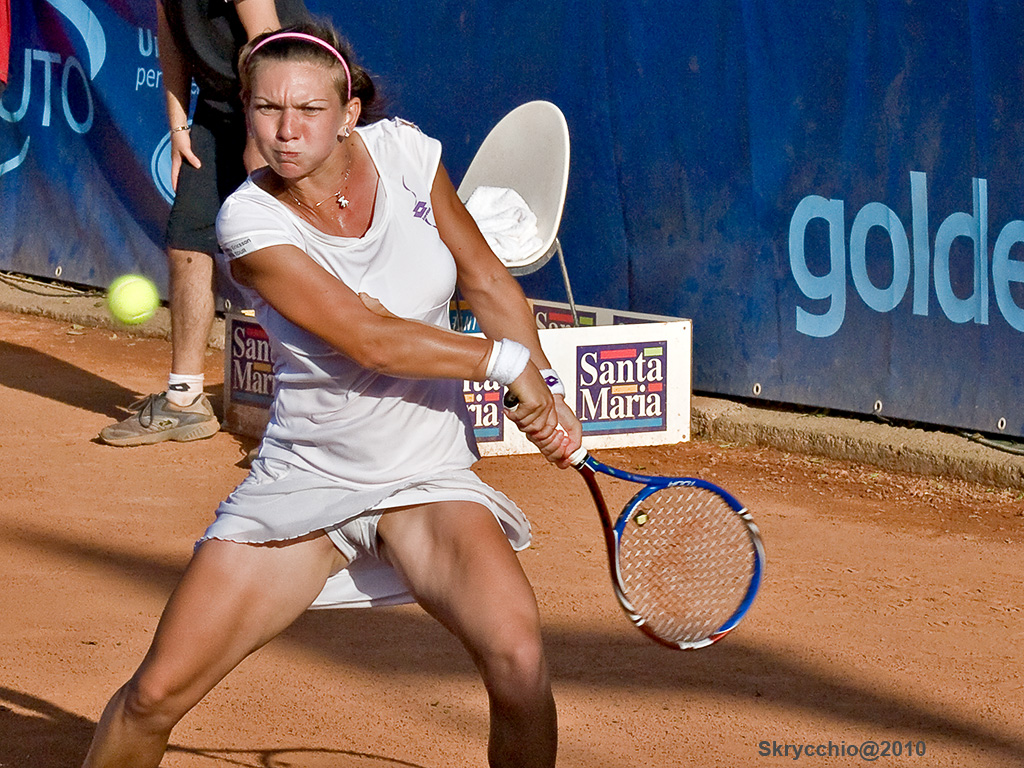The photograph captures a female tennis player mid-swing as she strikes a green tennis ball with her blue racket. She is wearing a white tennis outfit that consists of a t-shirt and a short skirt, along with white sweatbands on both wrists. Her stance is intense and focused, with her eyes narrowed and fixed on the ball. The background features a blue canvas banner with parts of the words "GOLDEN" and "UTO," which frame the player. Behind her stands a ball boy in black clothing and dirty sneakers, next to a white chair inside a white box labeled "Santa Maria." They are playing on a reddish-brown clay court under what appears to be a bright, sunny day. In the bottom right corner of the photograph, there is a watermark with the slightly transparent gray letters reading "SKRYCCHIO 2010."